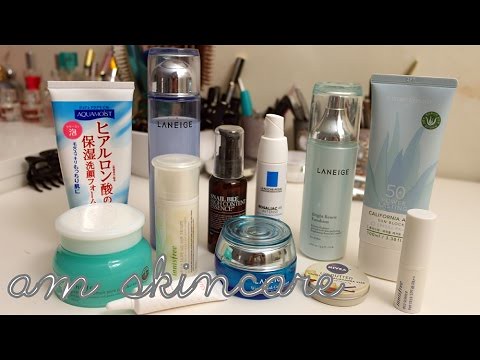The photograph features an intricate display of various skincare and makeup products, arranged meticulously as if prepared for a professional photo shoot. At the bottom of the image, a series of beauty products are lined up, with elegant cursive text overhead that reads "Anne Skin Care." Starting from the left, there's a tube adorned with Japanese writing. Below this tube, a jar with a white cap is visible. 

Next to the jar is a clear bottle labeled "Laneige," and positioned in front is an all-white bottle with a matching cap. Beneath these items, a tube rests at the bottom of the photograph. Centrally placed among the lineup is a prominent red spray bottle, flanked to the right by a white bottle featuring a blue square. In front of these, a blue jar with a silver lid draws the eye.

Further to the right, another spray bottle branded "Laneige" stands, and below it, a small compact marked "Nivea" is present. Continuing to the right, a blue squeeze bottle is observed, accompanied by a white stick resembling a lipstick container placed in front. The background reveals an array of hair and makeup accessories, adding depth and context to the comprehensive beauty arrangement.